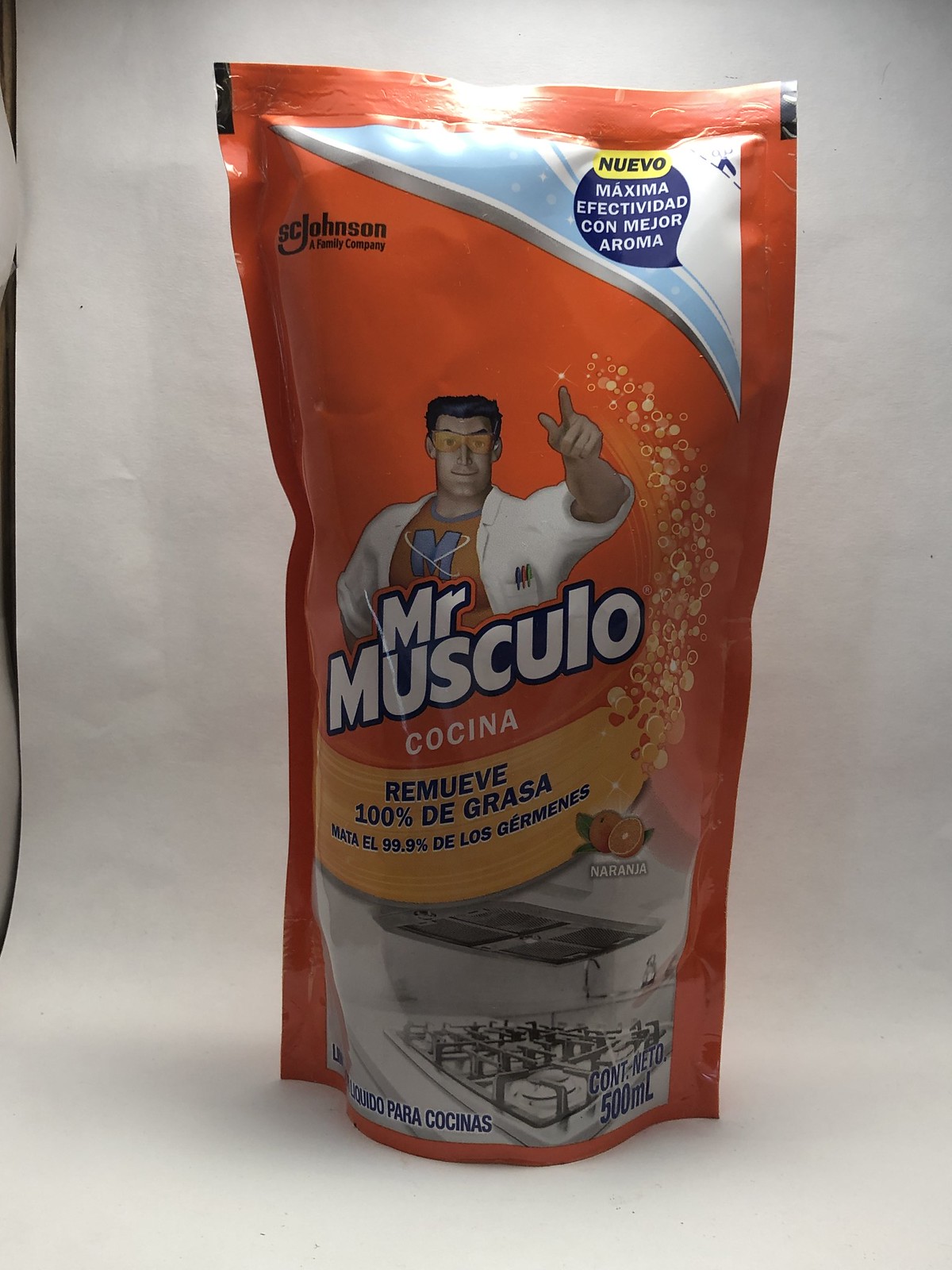The image showcases a cleaning product called Mr. Musculo Cocina, manufactured by S.C. Johnson. The product is packaged in a tall, orange, sealable plastic bag, similar in structure to a potato chip bag but with a flat, circular base for stability. The background of the photograph is a white sheet of paper that curves upward to form a seamless backdrop, although the upper left edge reveals a bit of a black strip beyond the paper.

The central graphic on the packaging features a man depicted from the waist up, with short, dark hair and an orange eye protector. He is dressed in a white lab coat over an orange T-shirt emblazoned with an "M." The man is pointing upward with his left hand, and a stream of white bubbles emanates from his finger, curling to the right before heading downward. Positioned prominently below the man, the product name, "Mr. Musculo," is written in bold white letters, followed by "Cocina" in smaller white text.

The packaging also includes several other elements: In the upper left corner, it bears the S.C. Johnson logo in dark navy lettering. On the upper right, there's a light blue and white triangular cut-out with a blue circle stating, "Maxima Effectividad Con Mejor Aroma" in white text, and above this, a yellow strip with "Nuevo" written in blue. Further down, a yellow curvy strip reads "100% De Grasa," indicating its grease-removal efficacy. At the bottom of the package, there's an image of a stovetop with burners, reinforcing the product's intended use in the kitchen. The bottom right corner notes the product volume, 500 ml.